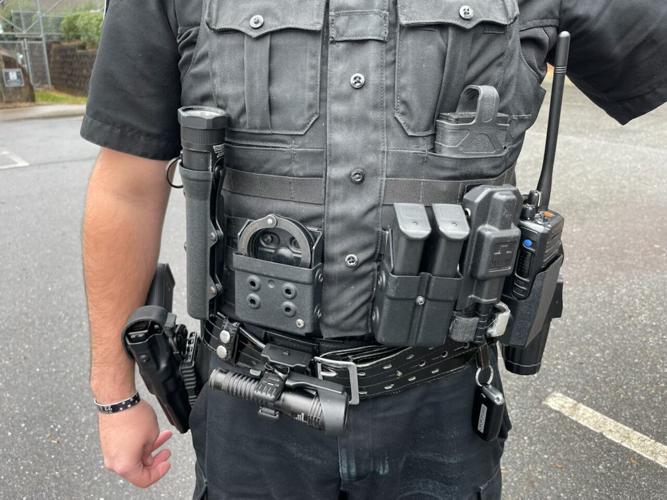This color photograph illustrates a detailed close-up of a law enforcement officer or security personnel seen outside during the day in a parking lot, which is identifiable by the white parking lines visible on both the right and left sides of the paved street. The focus is on the torso of the individual, who is dressed in tactical black clothing: a short-sleeved shirt and pants, complemented by a gray tactical vest featuring multiple pockets and gray buttons. The black belt with a silver buckle is loaded with essential equipment: a pistol in a holster on the left, a radio on the right, a flashlight, handcuffs, and what appears to be spare batteries or cylindrical objects, possibly another flashlight. The right side of the belt also has a keychain, and a black and silver bracelet adorns the officer’s right wrist. The overall detailed attire, which includes tasers and other gear, suggests the individual is involved in some level of law enforcement or private security work.